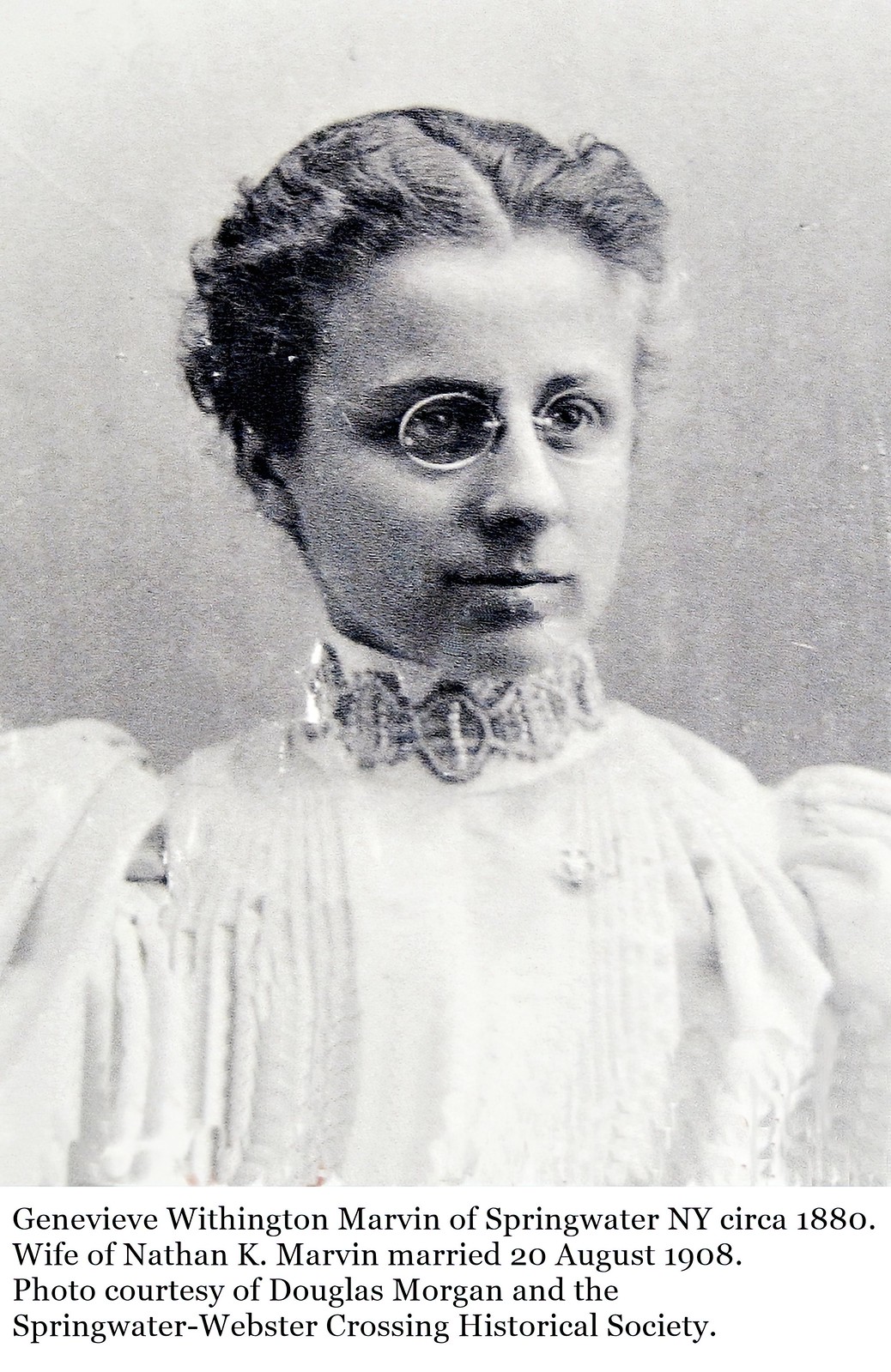This black and white photograph, likely taken circa 1880, showcases a young woman in her early 20s named Genevieve Withington Marvin from Springwater, New York. She is depicted from the mid-torso up, attired in a white Victorian-style chiffon or lace dress with puffy, fluffy sleeves and a high collar adorned with intricate beadwork. Her rounded face framed with short, combed-back dark hair, parted in the middle, features delicate wisps around her temples and ears. She wears thin, circular wireframe glasses and gazes contemplatively to the right. A distinctive brooch graces her neck, adding to her poised elegance. The photograph's backdrop transitions from darker gray at the bottom to lighter at the top. Text beneath the image identifies her as the wife of Nathan K. Marvin, whom she married on August 20, 1908. This photo, credited to Douglas Morgan and the Springwater Webster Crossing Historical Society, preserves a vivid glimpse into a bygone era.